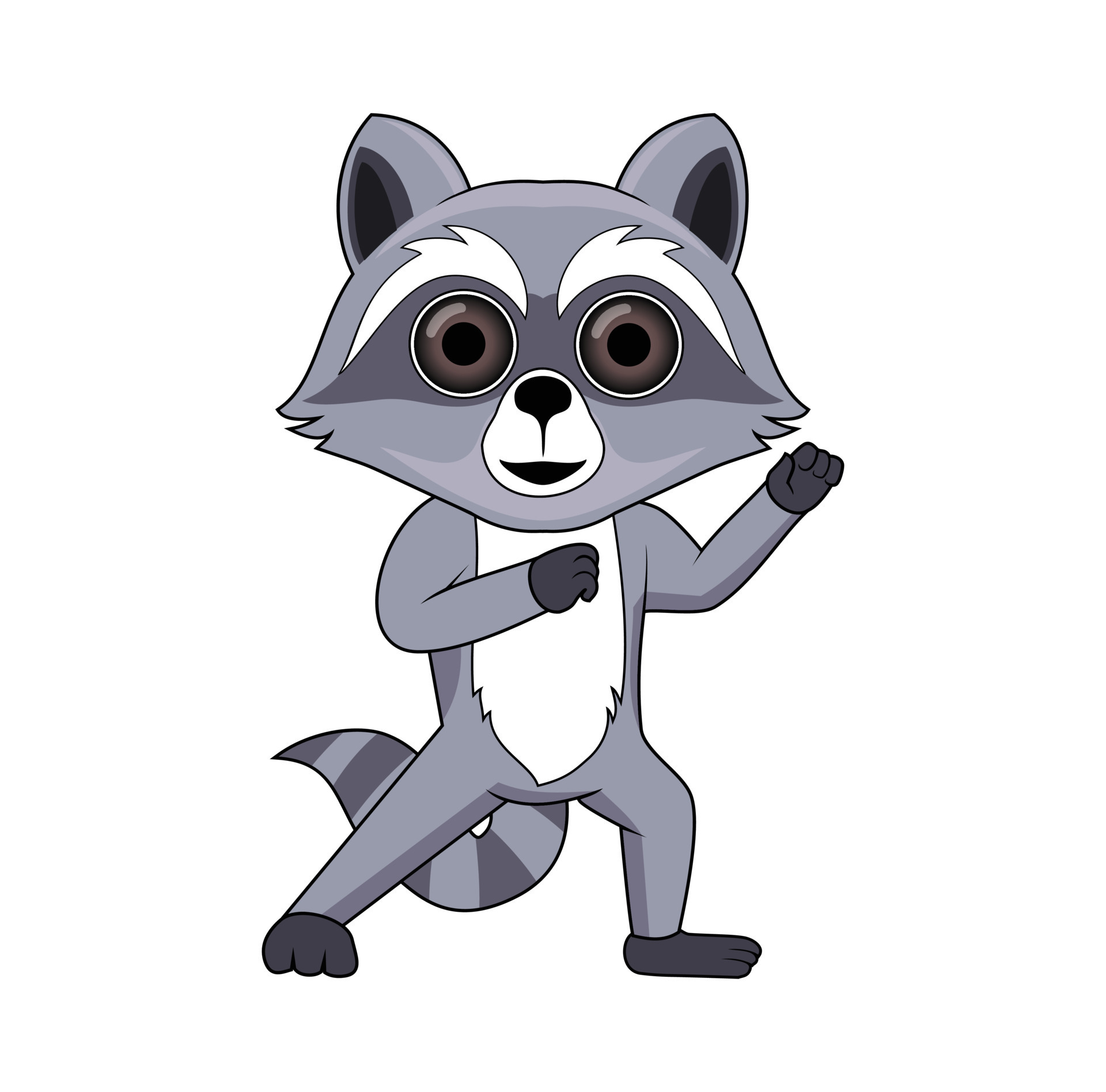This is an artistically rendered, cartoon image of a raccoon standing upright on its hind legs against a white background. The raccoon, drawn in a humanoid style, is looking directly at the viewer with a small smile and large, expressive brown eyes surrounded by a dark gray mask that accentuates its gaze. Its white bushy eyebrows and fluffy cheeks add to its animated appearance. The raccoon has a distinctive color pattern: gray ears with dark gray and black insides, a black nose and mouth, and a white area surrounding its nose and mouth. Its chest and torso are predominantly white, contrasting with the gray fur that covers the rest of its body. The raccoon's hands and feet are dark gray to black, and it holds its fists up in a pose that exudes confidence. Notably, it has a fluffy, gray and white striped tail that curls slightly behind it, contributing to its endearing and lively character design.